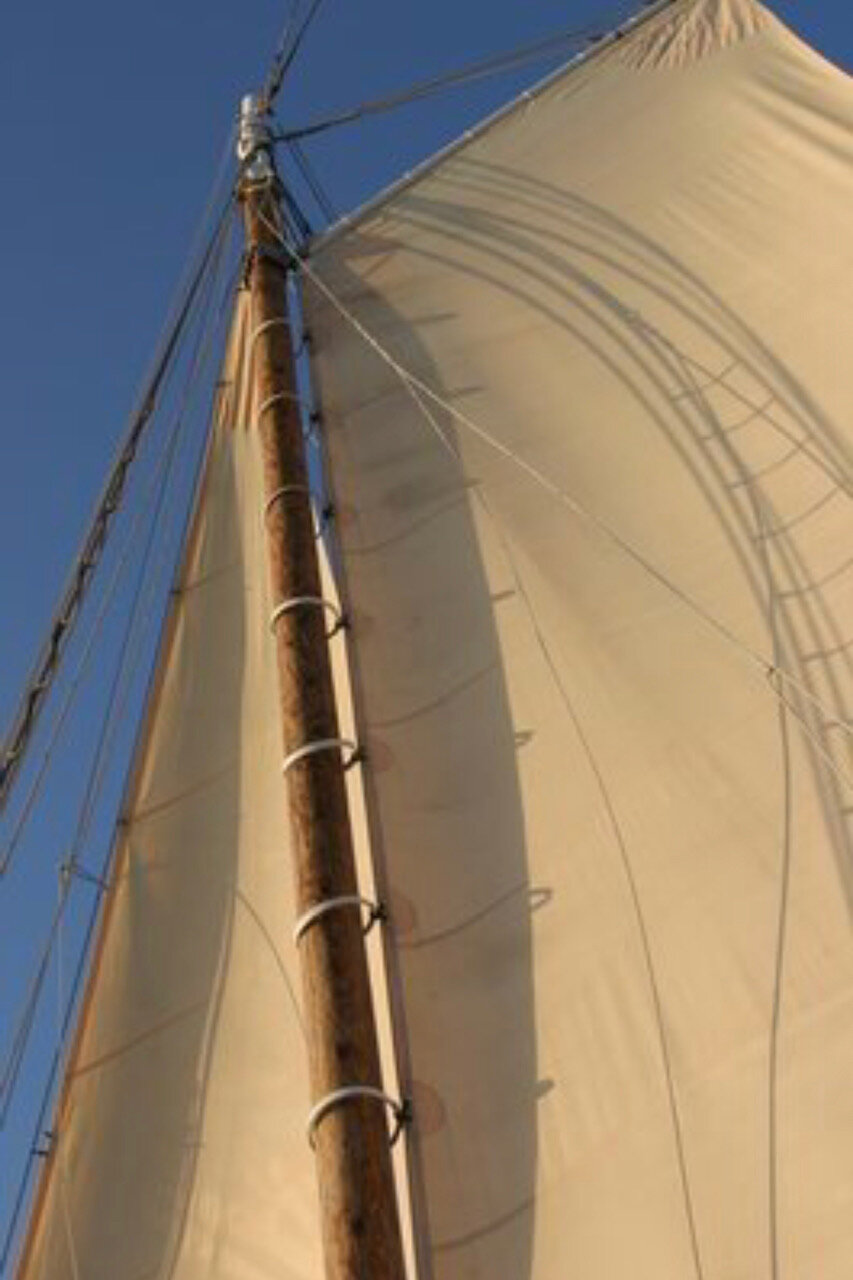This image captures a detailed and dynamic scene of a sail on a ship, likely an older vessel, as it moves through clear evening skies. The focal point is the ship's unpainted, wooden mast, adorned with metal rings which secure the sails. Two sails are visible: the larger, rectangular sail on the right, taut and full of wind, and a smaller, triangular sail on the left, both working in tandem to propel the ship. The sails are illuminated by a light source from the left, casting long shadows that emphasize the late hour of the day. Numerous ropes extend from the top of the mast, essential for hoisting and adjusting the sails. The sky in the top left is a deep, clear blue with no clouds, adding to the serene maritime atmosphere of the image.